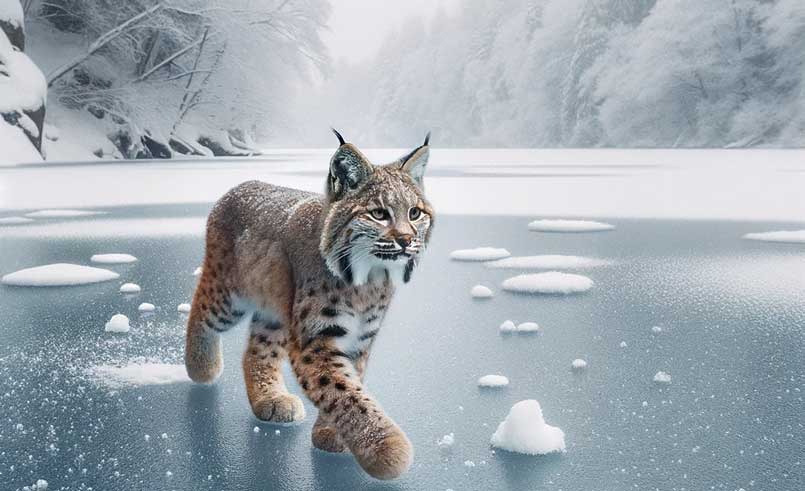This highly detailed AI-generated image depicts a young bobcat walking across a partially snow-covered, frozen lake in the dead of winter. The bobcat, moving toward the right of the frame, is meticulously rendered with black tufts of hair on its signature pointed ears, a brown to beige coat, and a dusting of snow along its back. Black spots decorate its chest and legs, while dark brown stripes extend from its eyes down the sides of its face. The ice, a slate blue color, is dotted with patches of powdery snow, and the lake's snow-covered banks are lined with many trees, some growing up a hill in the background. These trees and the foliage are heavily blanketed in snow, contributing to the scene's wintry atmosphere, with a white sky and a faint snowy mist hanging in the air.